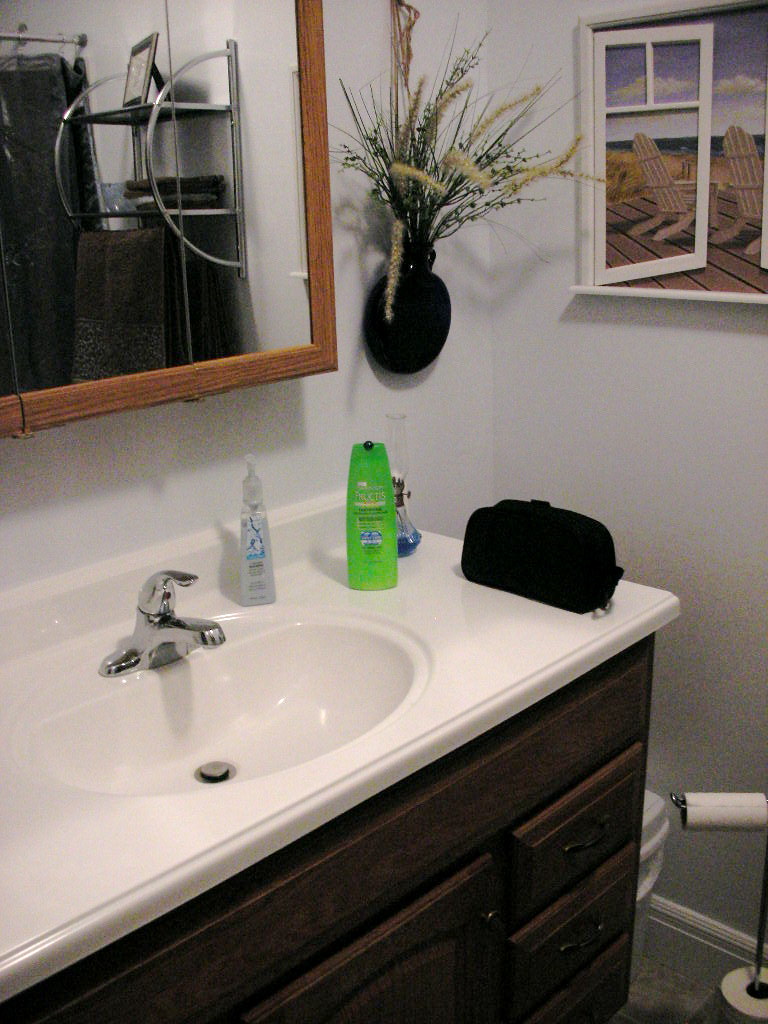A detail-rich photograph captures a corner of a bathroom with an intriguing mix of elements. On the upper right wall, a highly realistic painting depicts an open window overlooking Adirondack chairs on a deck by the ocean, designed to look like a real window swung open to the left. The walls are painted a pale gray or white. In the bottom right corner stands a sleek, chrome freestanding toilet paper holder, boasting a nearly full roll on its arm and an additional roll stored vertically.

Barely edging into the frame, the closed lid of the toilet is visible. Above it, a pocket vase with dried flowers and grasses adds a touch of rustic charm. Adjacent to this, on the larger wall coming together at a corner, hangs a framed mirrored medicine cabinet. This seems to function with doors on either side that reveal interior shelving.

A white countertop with a built-in sink features a chrome faucet with a single handle. Various toiletries adorn the countertop, including a Garnier Fructis shampoo bottle, a black cosmetic bag, and a clear, square-shaped liquid hand soap dispenser, reminiscent of Bath and Body Works packaging. The dark wood vanity supporting the countertop has a vintage feel, highlighted with pull handles.

Reflected in the mirrored cabinet, a chrome hotel-style shelf is visible, mounted on an unseen wall. This shelf has two tiers: the top one displays a framed picture with a kickstand, while the bottom shelf holds a neatly folded dark brown hand towel and more towels. The reflection also hints at a dark shower curtain hanging from a rod, completing this slice-of-life snapshot of a meticulously detailed bathroom corner.